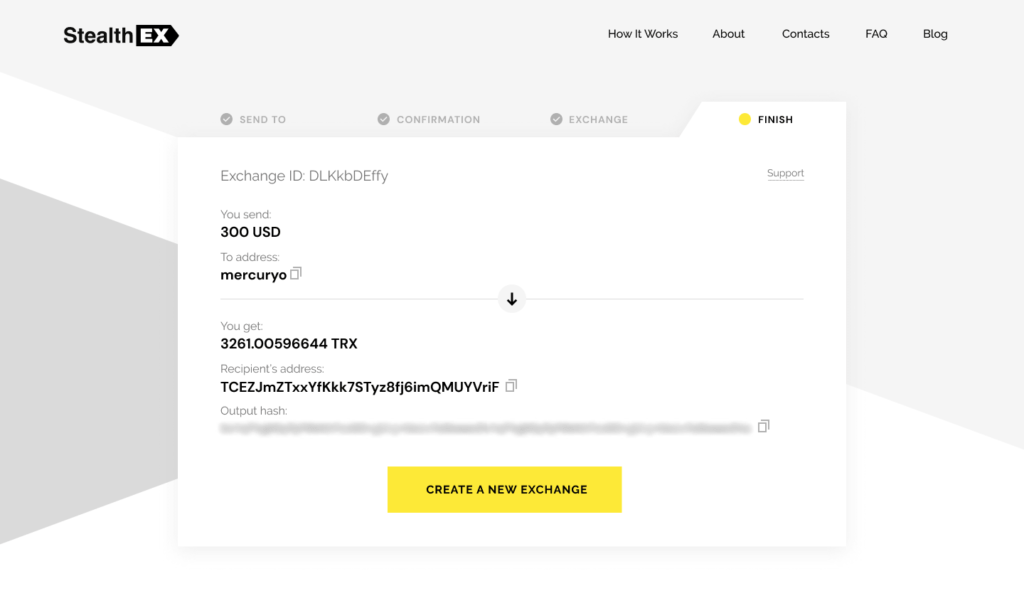The webpage for Stealth EX features a navigation bar at the top right with tabs labeled "How it Works," "About," "Contact," "FAQ," and "Blog." 

In the main section of the webpage, the exchange process is outlined with a series of steps:
1. **Send To** - Indicated by a gray circle with a white checkmark.
2. **Confirmation** - Also marked by the same checkmark icon.
3. **Exchange** - Followed by the same checkmark.
4. **Finish** - The current step being displayed.

Below these steps is the **Exchange ID**: "DLKKBD_EFFY." To the right, there is a **Support** link.

Further details include:
- **You Send**: $300 USD
- **To Address**: "Mercurio," accompanied by a Documents icon.
- A thin light grey line with an arrow pointing to the result:
- **You Get**: 3261.00596644 TRX

Following this is the **Recipient's Address**: "TCEZJmZTzxxYfkkk7STyZ8fj6imQMUYVriF," with another Documents icon next to it.

At the bottom of the page, there is a **Create a New Exchange** button for initiating a new transaction.